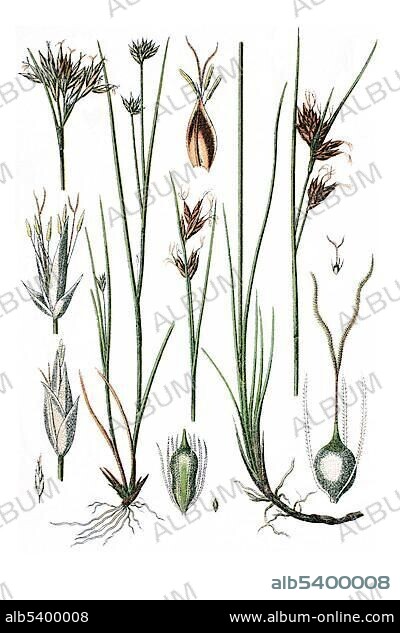The image showcases various grass drawings, standing out against a white background marked with numerous diagonal gray "album" watermarks. The plants range from simple green stems and subtle purple flowers to more intricate systems, with some illustrations extending to show distinctive root structures, including a garlickish-looking bulb. A small black rectangle stretches across the bottom of the print, displaying "ALB 5400008" on the left and "www.album-online.com" on the right. The serial number "5400008" also appears in sage green above the rectangle. The overall composition presents a subdued palette of greens, browns, and light tans, highlighting the botanical details without any dirt backdrop.